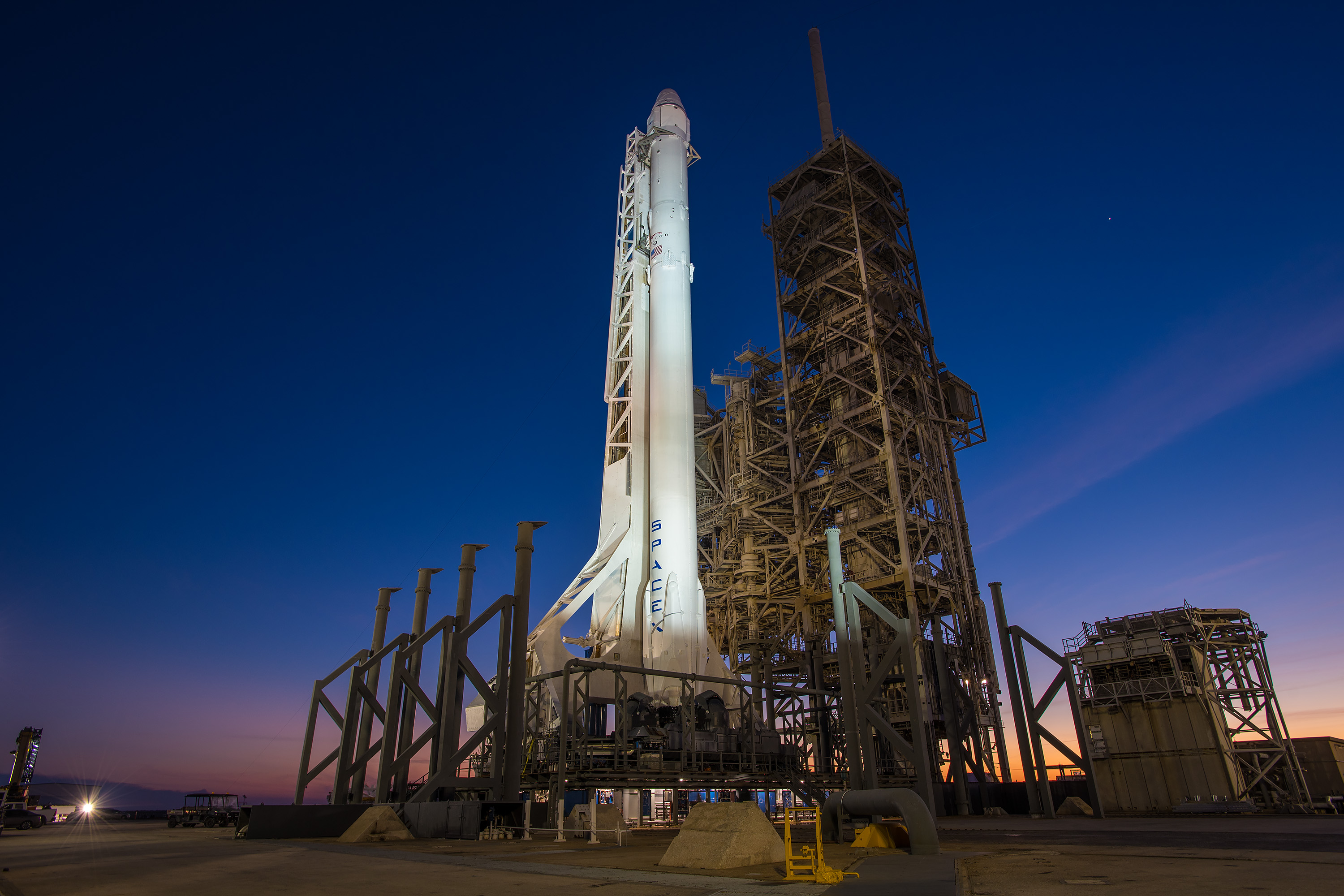In this photograph, a tall and narrow SpaceX rocket stands prominently on a launch pad surrounded by various support structures and equipment. The rocket is illuminated against the backdrop of a deep blue sky, indicating that the photo was taken at dusk or early morning. The word "SpaceX" is clearly visible on the white body of the rocket. The launch site is well-lit, highlighting a metal scaffolding structure to the right of the rocket which supports its impressive vertical height. Additional elements include concrete blocks, various metal poles, and a spotlight in the distance. There is also a small vehicle, possibly a yellow dolly, and what appears to be a metal building beside the scaffolding structure. Far off on the left side of the image, a helicopter can be seen hovering, adding to the scene's dynamic energy. The entire area is bathed in artificial light, contrasting with the natural colors of the early or late day sky.